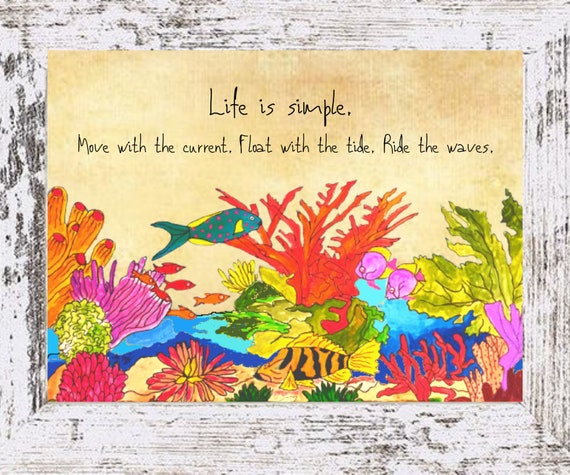The image is a vertically framed cartoon drawing with a rustic driftwood frame that has a weathered mix of white, gray, and blotches of black. The frame surrounds an underwater scene featuring various colorful aquatic plants and corals. The background is a subdued light brown, almost beige, giving the entire image a soft, muted appearance. At the top of the image, thin white letters spell out the phrase: "Life is simple, move with the current, float with the tide, ride the waves." Below this phrase, a vibrant coral reef is illustrated, showcasing diverse marine life. You can see an orange and black striped fish, two pinkish fish, a blue fish with small purple dots, and additional small orange and pink fish. The water is depicted in turquoise hues, adding to the overall serene aesthetic of the piece.